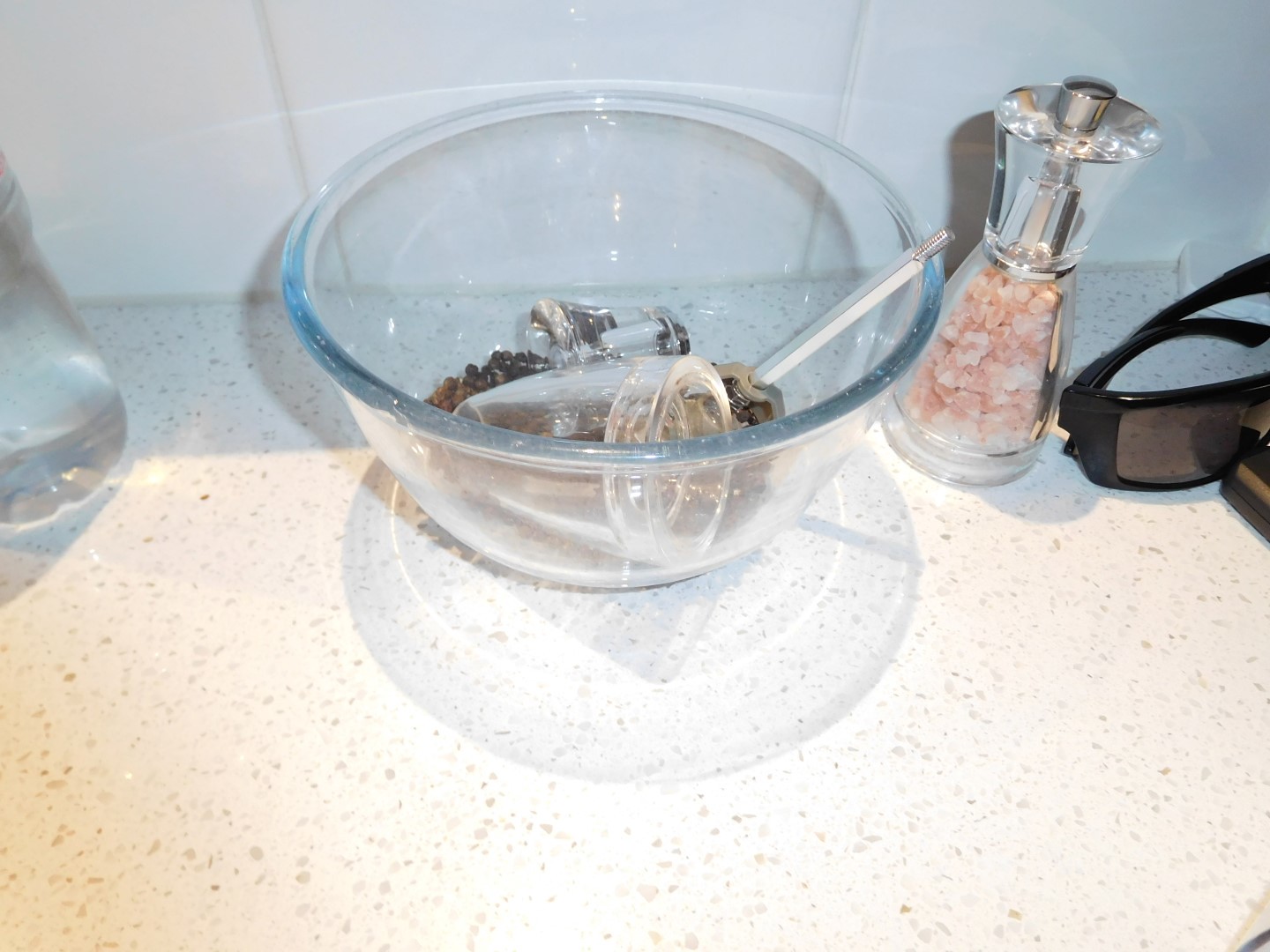A pristine, white kitchen countertop is centered against a clean, white back wall. On the countertop, a clear glass bowl occupies the middle, filled with various small glass items and metal bolts, adding a touch of eclectic charm. To the right of the bowl, a glass salt shaker filled with pink Himalayan salt stands out, while nearby, a couple of clear drinking glasses sit neatly arranged. To the left, a simple white container adds to the organized aesthetic of the kitchen space.